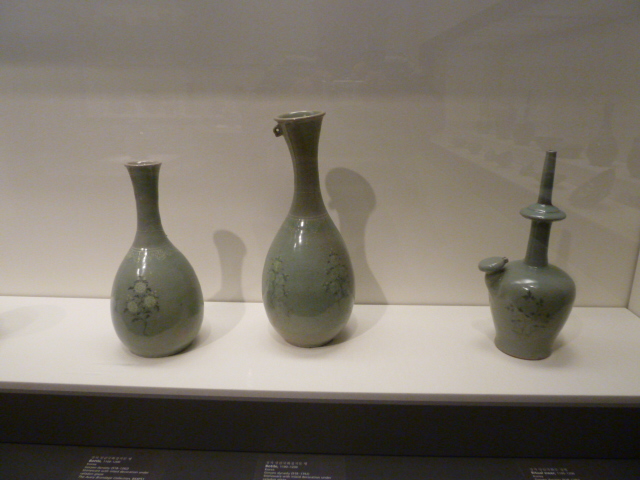This photograph captures a museum display case showcasing three distinct pieces of grayish-brown pottery on a white shelf against a similar-colored wall. The serene, reflective sheen on the vases suggests they are glazed ceramics, each adorned with intricate floral patterns. Arranged from left to right, the vases vary in shape and size, creating a harmonious yet diverse visual. The first vase features a simple oblong shape tapering to a rounded opening, beautifully decorated with a white three-blossom floral design. The middle vase, slightly taller and wider, includes a small loop near its opening, possibly meant for threading a wire or string. The third vase, more intricate and unique, displays a bulbous base with a circular valve on the side and a central spire extending upwards, adorned with a circular disk midway. Each vase casts a soft shadow, enhancing the depth of the display, and in front of them, black placards with unreadable white text likely provide historical context and descriptions. A faint reflection in the glass cover adds a subtle layer of depth to this meticulously curated exhibit.